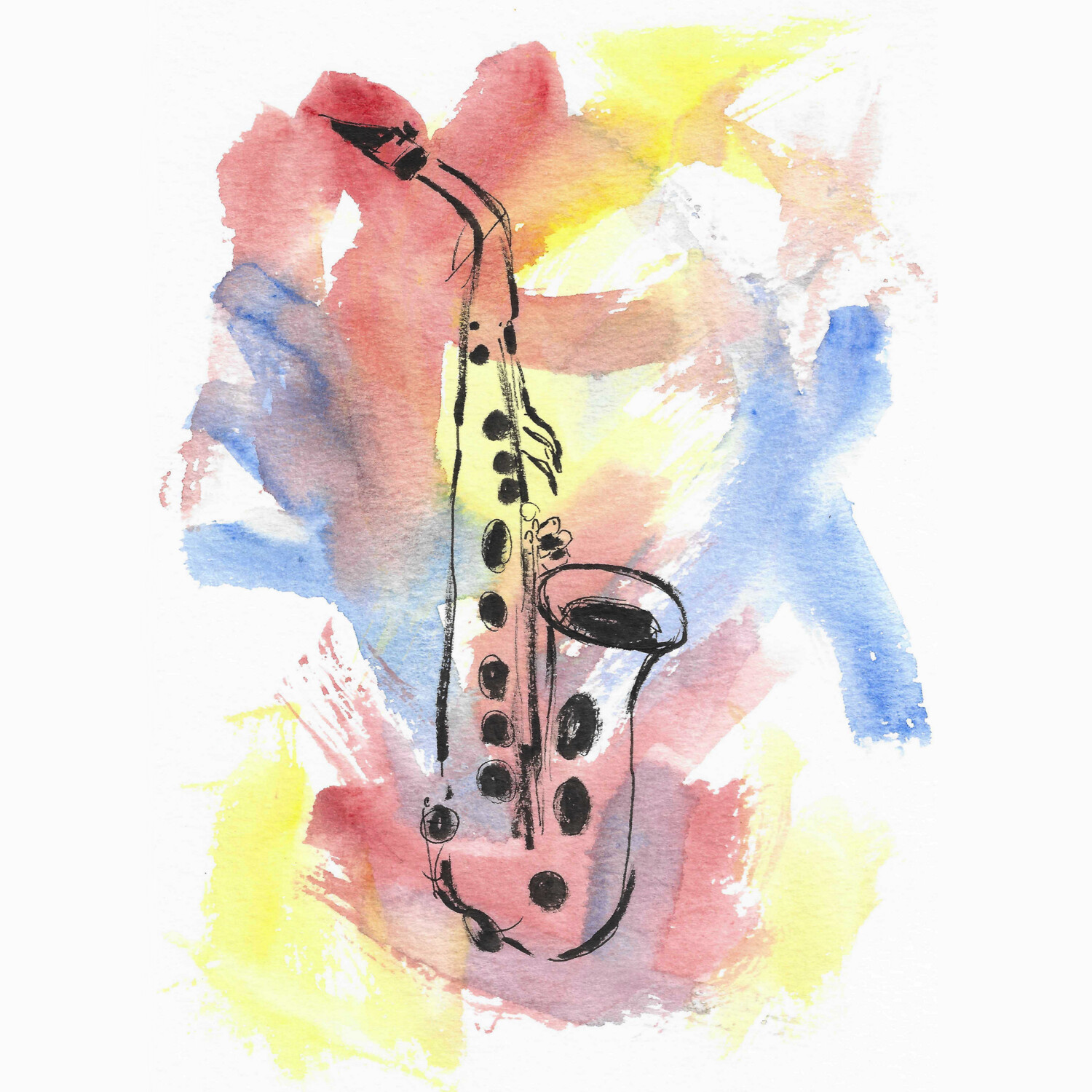The rectangular painting features a slightly off-white background adorned with vibrant watercolor strokes of red, yellow, and blue that appear haphazardly spread across the canvas. Prominently displayed in the center of the composition is a roughly drawn saxophone, executed in black. The saxophone, illustrated from the mouthpiece down to the flared bell, is outlined with a bold black line that makes it discernible despite the abstract nature of the entire piece. Each individual key of the saxophone is meticulously painted in black, allowing for detailed recognition of the instrument's components. The mouthpiece and bell are clearly defined, with the black opening of the bell standing out. The colorful background, consisting of broad and random paint strokes, adds a dynamic contrast to the central black saxophone, which is depicted with a slight silver tint, highlighting its complex mechanism. The painting exudes a sense of abstract whimsy while maintaining the recognizable shape and details of the saxophone.